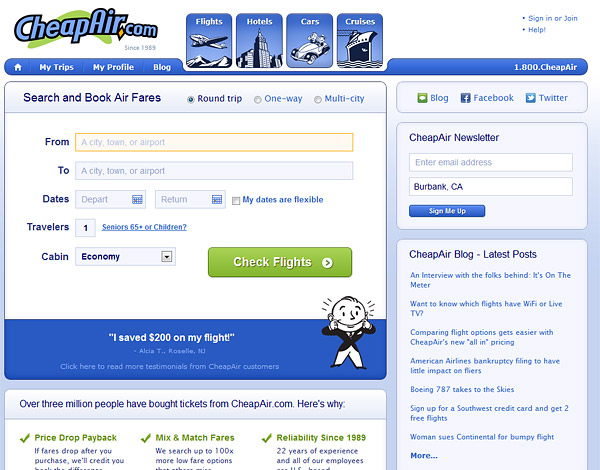![CheapAir.com Screenshot](link_to_image)

The interface of CheapAir.com is showcased in this detailed image. At the top, the website's logo is prominently displayed in blue lettering against a green background. Below, four main icons for Flights, Hotels, Cars, and Cruises are featured, each accompanied by a distinct ink-style drawing: an airplane for Flights, towering buildings for Hotels, a vintage Monopoly-style car for Cars, and a classic black and white cruise ship for Cruises.

The central area of the page is devoted to searching and booking airfares, complete with fields for the departure city, destination, travel dates, flexible date options, number of travelers, and traveler details like seniors or children. The default cabin setting is Economy, with a dropdown menu available for other options. Once all the necessary information is entered, a green button enables users to check flight availability.

A highlighted section at the bottom features a testimonial by Alicia T. from Roselle, New Jersey, who saved $200 on her flight. Accompanying the testimonial is a black-and-white hand-drawn illustration of a smiling figure. Additionally, the site's credibility is emphasized with a note that over 3 million people have purchased tickets from CheapAir.com, benefiting from features like Price Drop Payback, Mix and Match Fares, and reliability since 1989.

On the right-hand side, the Cheap Air newsletter signup section invites users to enter their email address and subscribe. This section also features a blog feed with various posts including interviews, tips on flights with Wi-Fi or live TV, comparisons of flight options, updates on American Airlines' bankruptcy filing, the inaugural flight of Boeing 787, and a legal case involving a woman suing Continental for a bumpy flight. 

Overall, the website is designed to be a comprehensive travel booking platform with user-friendly tools and valuable customer testimonials.